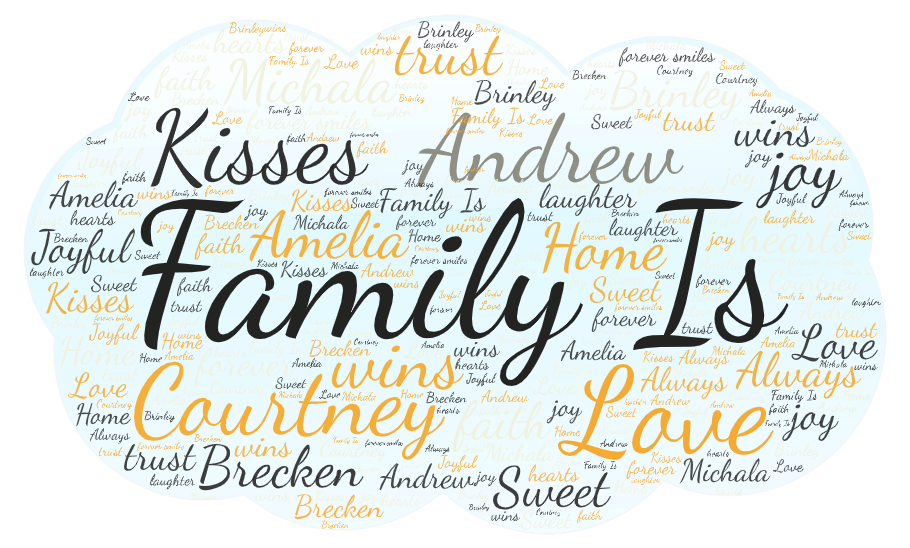This graphic features a visually captivating text cloud on a very light blue background, shaped like a rounded, scalloped cloud. The words are spread across the cloud in various sizes and colors, all in an elegant script font. The cloud is adorned with words such as "TRUST" in gold, "BRINLEY" in black, and "KISSES" overlaying "ANDREW" in lighter gray, prominently positioned in the center. The largest text in the middle reads "FAMILY IS" in black. Surrounding these central words are various other names and sentiments, including "WINS," "JOY," "LOVE," "AMELIA," "COURTNEY," "BRECKIN," "M-I-C-H-A-L-A," and more. The text runs in different directions but remains horizontal, creating a dynamic, lively pattern against the soft blue cloud shape. Additional words such as "JOYFUL," "SWEET," "HOME," and "ALWAYS" contribute to the overall theme of positivity and connection within the family context.